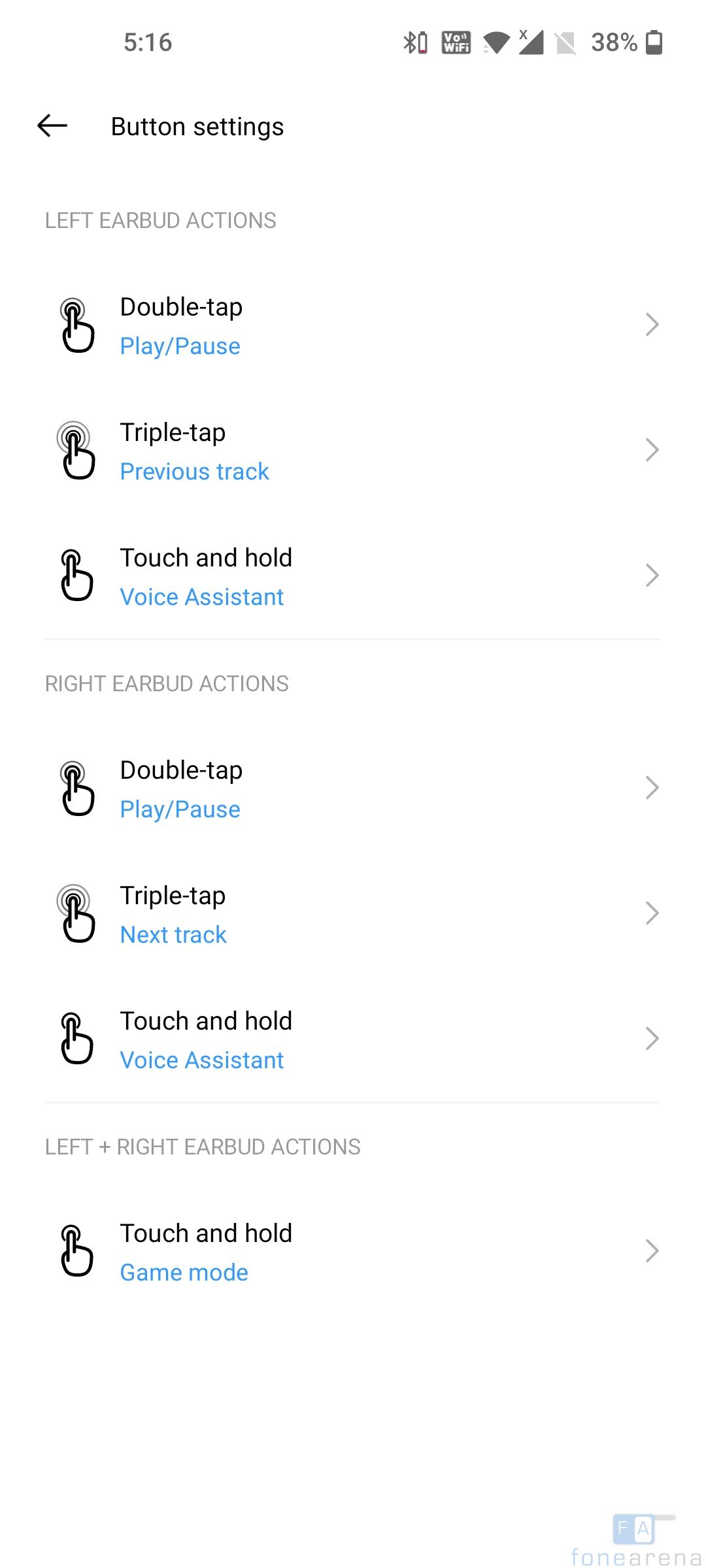The image depicts a settings menu from a smartphone, specifically for customizing the controls of wireless earbuds. The interface features a clean, white background with standard elements displayed at the top: the current time on the left, along with the Bluetooth symbol and battery percentage on the right. A black back arrow is positioned at the top left, indicating navigation back to a previous screen. The header reads "Button Settings."

Below this header, the screen is divided into two sections: "Left Earbud Actions" and "Right Earbud Actions." For the left earbud, the following actions can be configured:
- Double tap: Play/Pause
- Triple tap: Previous track
- Touch and hold: Activate Voice Assistant

For the right earbud, the actions are:
- Double tap: Play/Pause
- Triple tap: Next track
- Touch and hold: Activate Voice Assistant

Additionally, there is an action for pressing both earbuds simultaneously:
- Touch and hold: Activate Game Mode

At the bottom of the screen, the company logo and name are displayed: a blue and white "FA" logo, accompanied by the name "Fonarina," suggesting this is the brand behind the earbuds. The menu appears to be customizable, with arrows and options that likely allow users to adjust the functions for each button press.